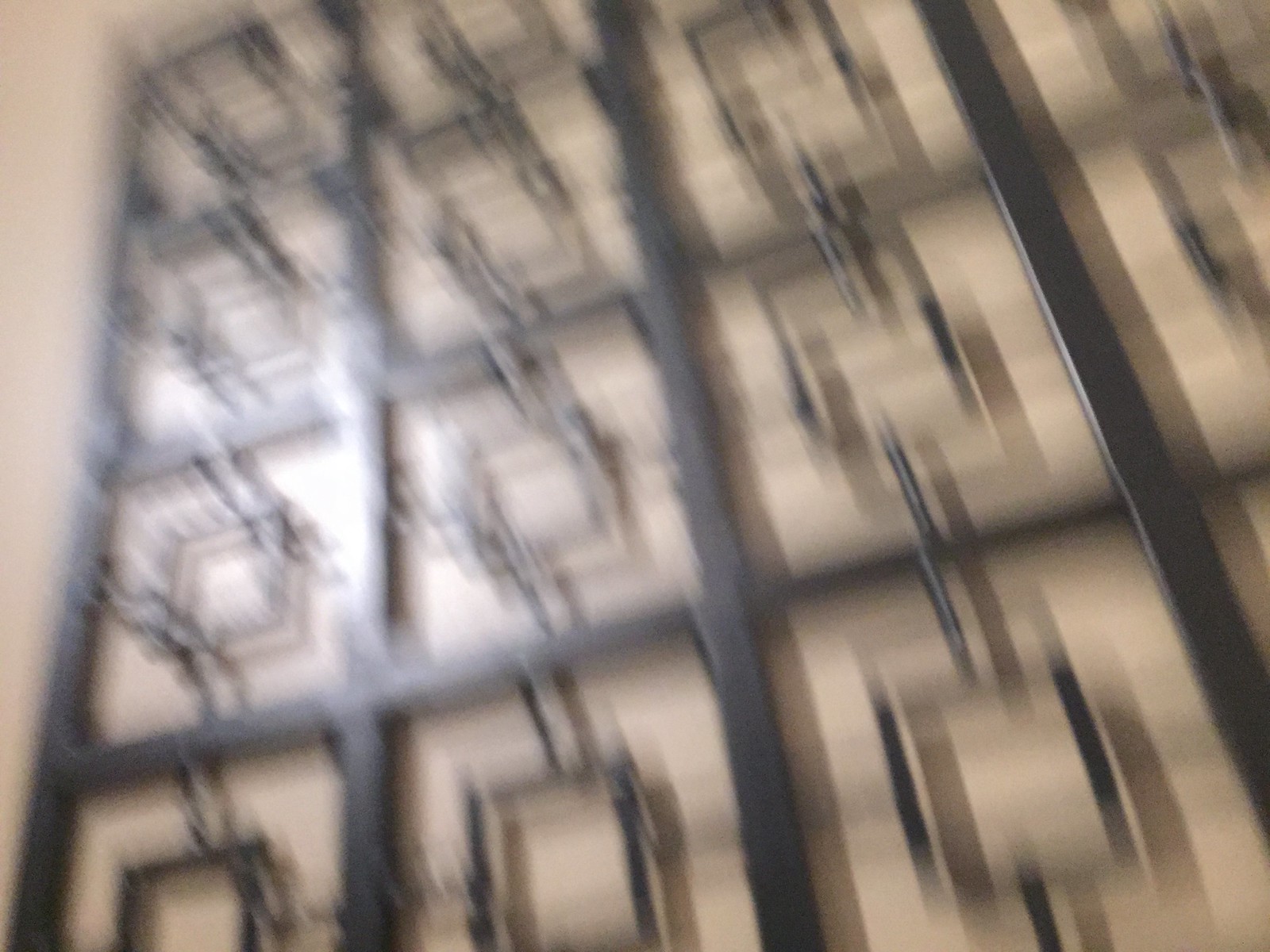This photograph, which is extremely blurry and out of focus, captures what appears to be a metal wall decoration. The pattern consists of a square grid made out of a dark brown or aged bronze metal frame. Within each larger square, there are smaller inner squares that are attached by thin metal rods centered on each side. These interconnected squares form a cohesive and intricate grid pattern that is placed against a beige or tan-colored background. The light source illuminating the photograph seems to be coming from the left-hand side, adding a subtle highlight to the wall decor and enhancing the contrast between the dark metal and the lighter background.